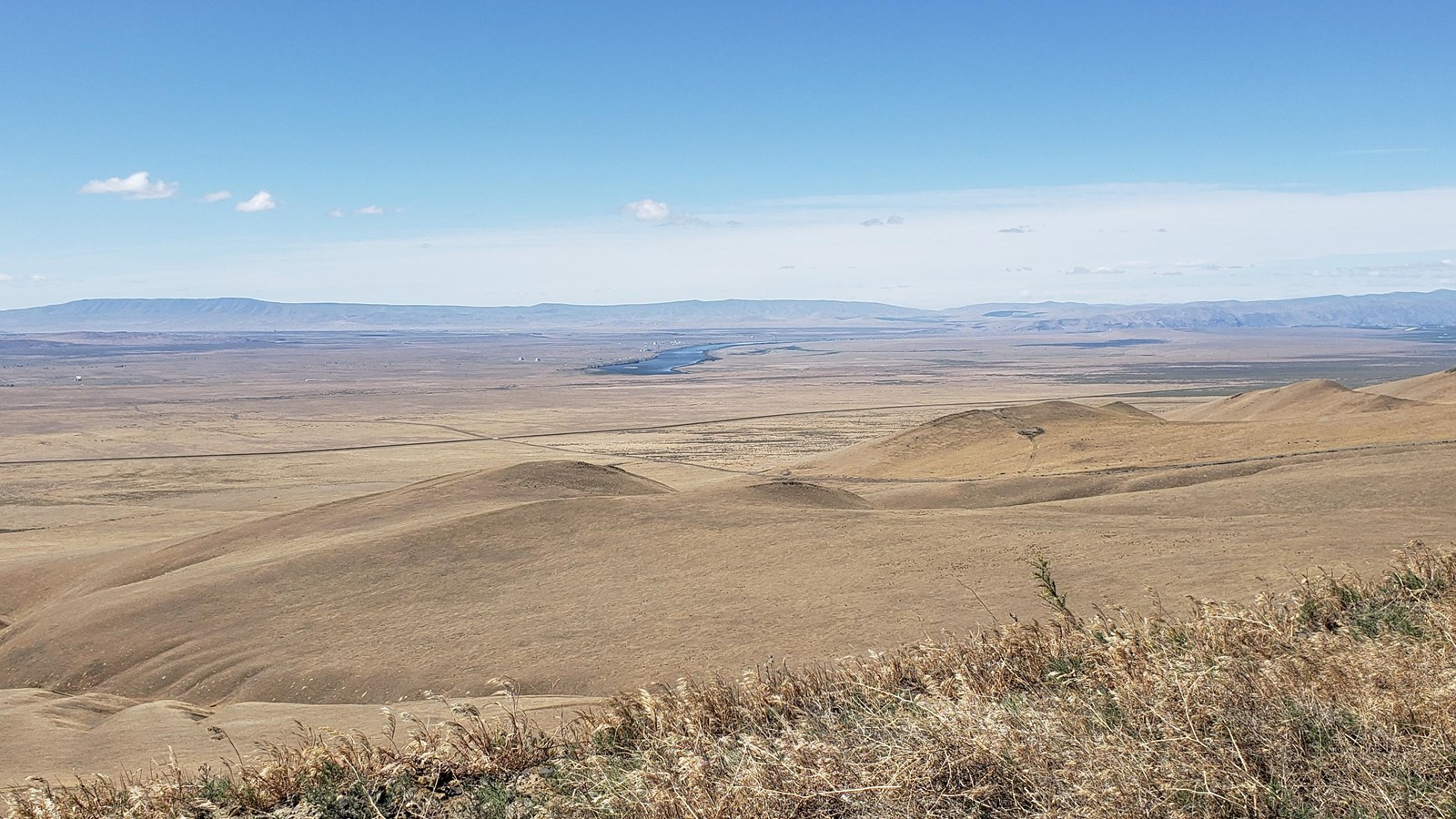The photograph is a detailed landscape taken during broad daylight, capturing the expansive, arid terrain from atop a grassy hill. In the foreground, dry grasses are visible, indicative of a prolonged lack of water. The vast expanse stretches out for miles, composed predominantly of low rolling hills covered with brown, dried-out grasses, evoking the characteristics of a desert or prairie. The middle distance features a noticeable divot or trench that adds texture to the land. Stretching towards the horizon, the landscape flattens, though the far edges reveal distant low mountains. Toward the center-right of the image, a body of water, possibly a river or lake, can be seen glistening under the bright sun. The sky occupies the upper third of the photograph, transitioning from a deep blue at the top to a lighter whitish blue near the horizon, dotted with a few scattered puffy white clouds. The scene is strikingly bright and sunny, with no significant cloud cover to diffuse the sunlight.